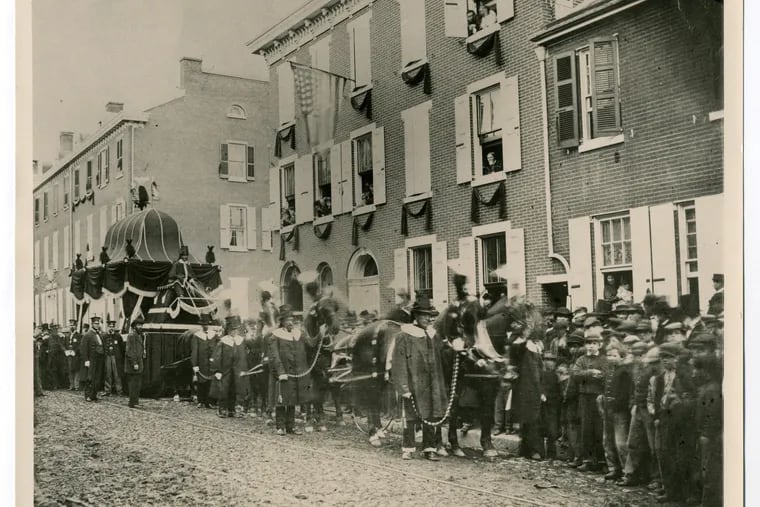This black and white vintage photograph, likely from the late 1800s or early 1900s, captures a bustling street scene during a parade. Men and boys, predominantly dressed in dark, long coats and hats, fill the sidewalk and street in front of a row of three-story brick buildings adorned with white outer window shades. Some windows are open, with onlookers peering out, adding to the lively atmosphere. An American flag hangs from one of the windows, further indicating a public celebration. Central to the image is a uniformed group of men guiding horses adorned with feathered headgear, pulling a stagecoach-like float with a covered area resembling a throne, likely to shield a dignitary or special guest from the sun. The photograph is square with grayish borders on the sides, and the throng of people extends from the lower right corner across to the left, just above the center, emphasizing the event’s scale and significance.